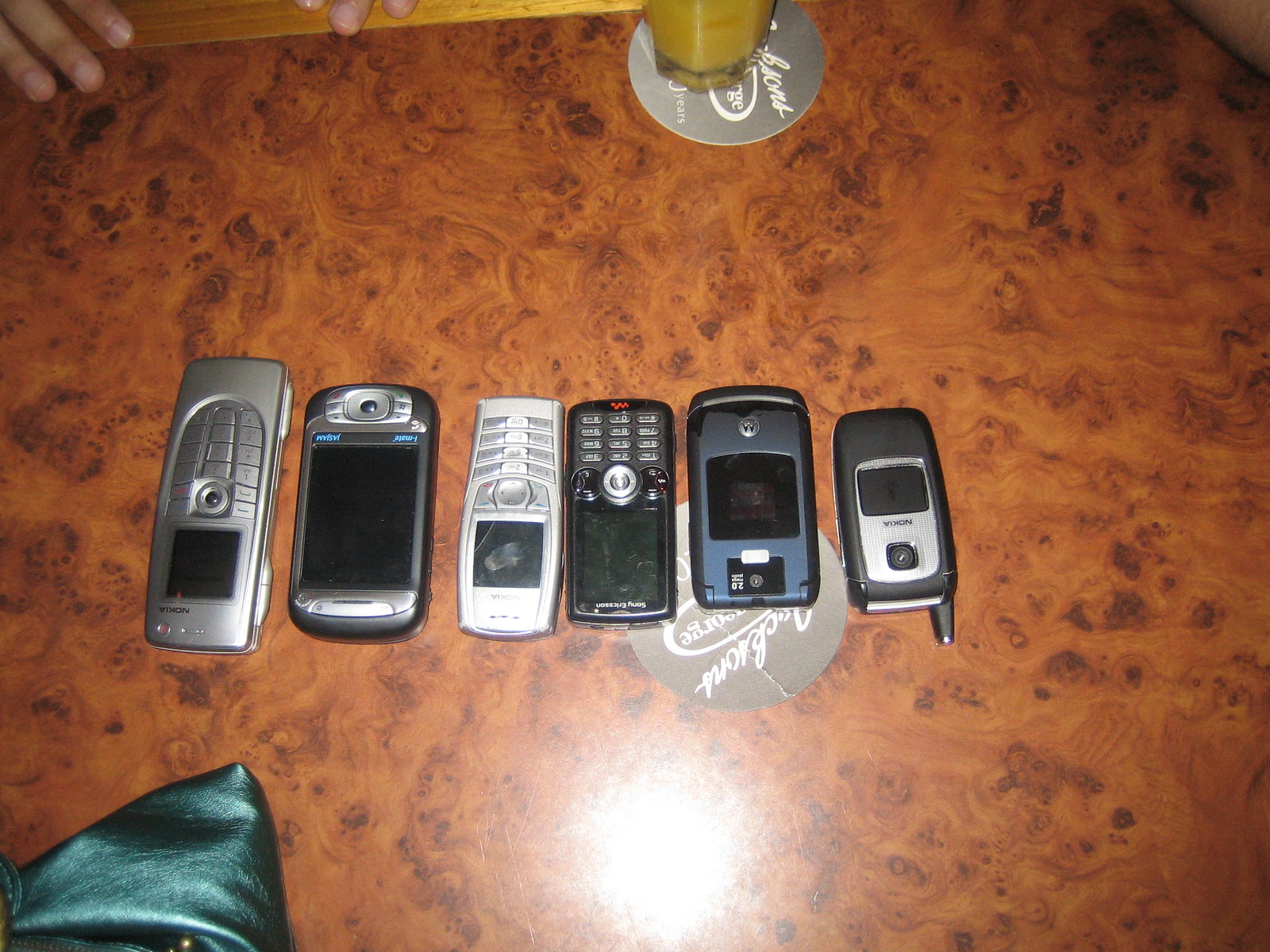An overhead photograph reveals six vintage mobile phones arranged on a brown marble table, captured from an upside-down vantage point, with the bottoms of the phones nearer the top of the image. The collection includes various models such as an old silver Nokia, a BlackBerry, a small Nokia with a number pad, a bluish Motorola flip phone, and another flip phone with a nubby antenna. A green piece of fabric, likely a metallic leather purse, is bunched up in the bottom left corner, while two gray coasters are also visible—one under two phones and another near the top center, possibly with a glass of liquid on it. The table's reflective surface adds a bright orb of light towards the bottom of the photo, and a pair of fingers can be seen peeking in from the upper left corner.